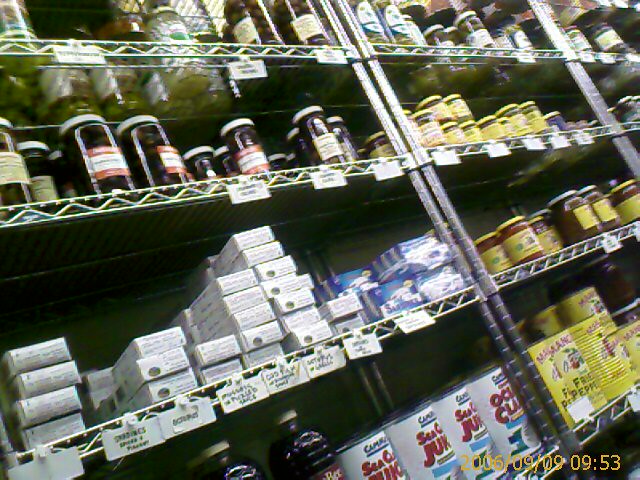The image depicts a warehouse-style store, characterized by three rows of metal racks filled with a diverse array of food items. The shelves, tilting counterclockwise from lower left to upper right, feature at least five levels of storage, brightly lit by overhead lighting. The most prominent racks hold a variety of bottles, jars, and cans. 

The rack on the left side is abundant with white, purple, and green packaged items, along with numerous bottle jars, some of which resemble salsa jars and olives, though the exact labels are too small to decipher. This rack also contains rectangular white boxes that might house personal care products.

The central rack prominently displays stacks of bottles and jars with yellow labels, some potentially containing Old El Paso tomato sauce or pickled items. Below these are larger jars with white lids and dark contents, as well as cans featuring seafood, clams, and fresh peppers. There are also sardine cans, the kind that require peeling open, situated on these shelves.

In the background, a glimpse of another rack can be seen, hosting an assortment of miscellaneous items. Small price tags dangle from the shelves, further emphasizing the industrial yet organized setting of this warehouse-type grocery store.